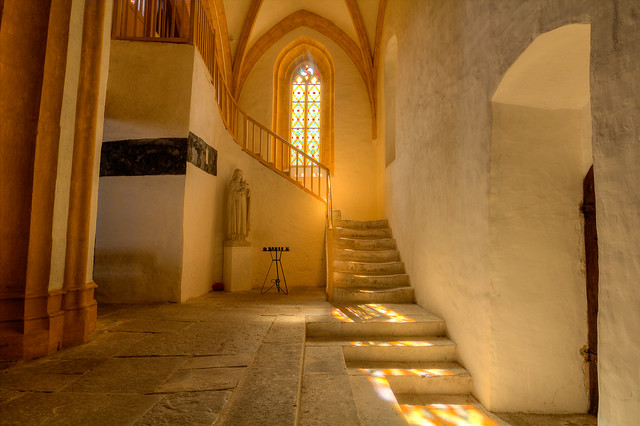This detailed photograph captures the warm, well-lit interior of an old stone building, with predominantly thick white and off-white walls. The floor is a mix of gray tile and stone, giving the room a sturdy yet elegant feel. On the left-hand side, wooden pillars ascend to the right, complementing the room's aesthetic. Central to the image is a striking white stairwell with a graceful wooden banister. This stairway curves up and spirals to the left, guiding the eye toward a charming stained glass window at the top, adorned with red and green dots and crossing patterns. The light filtering through this window casts a beautiful array of colored reflections onto the stairwell below, adding a magical touch to the scene.

To the right of the image, an archway leads to a door, though only a sliver of the wooden structure is visible. This doorway beckons curiosity, hinting at further architectural beauty beyond the frame. Below the staircase, a small black candle stand sits gracefully on the floor, accompanied by a stone cream statue, both adding to the quaint, historical ambiance. The walls to the left feature intriguing black markings, enhancing the room’s antique charm. This interior shot captures not only the intricate details but also the warmth and character imbued by natural sunlight filtering through the stained glass, creating a harmonious blend of history and artistry.